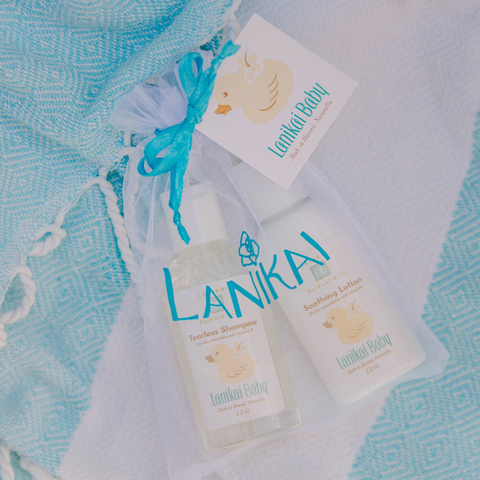The photograph showcases a gifting bundle of baby care products, prominently featuring two bottles housed in a see-through mesh bag. The bottles are neatly wrapped and tied at the top with a blue ribbon, accentuated by a white tag adorned with a yellow duck and blue text reading "Lanikai Baby." The left bottle is labeled "Tearless Shampoo" with subtle writing below that is difficult to decipher, except for the brand name "Lanikai Body." The right bottle is marked as "Soothing Lotion" and similarly features the "Lanikai Body" brand name. Both bottles carry the same yellow duck motif and have undecipherable small text, possibly indicating the volume. They are displayed against a backdrop of a textured, light blue knitted blanket, intersected diagonally by a white cloth. The setup suggests a cozy, nurturing theme suitable for baby-related products.